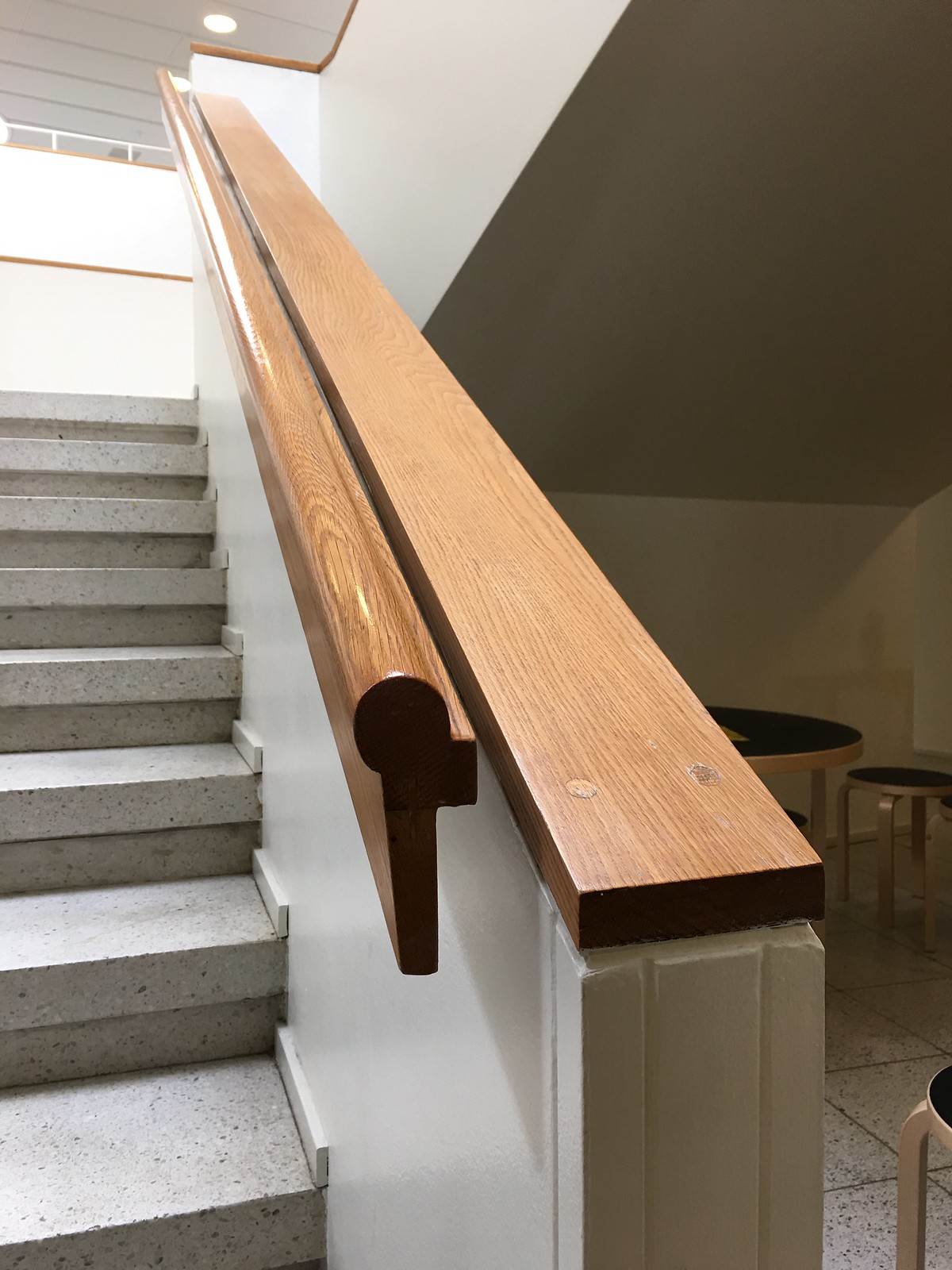The image showcases a sleek staircase made of light grey concrete steps. These pristine stairs lead up to an eloquent hall adorned with a broad window, letting in ample natural light. The main attraction is the sturdy, smooth wooden handrail crafted from solid oak, featuring a polished, medium-brown wood grain. It boasts a flat elongated wooden board following the top curvature, enhancing both style and grip with its robust, flat base and rounded edge. The lack of carpeting on these smooth steps makes them look particularly slippery, potentially hazardous when wet.

Adjacent to the staircase, on the right side, there is a small alcove with a black metal table accompanied by matching benches and a stool, resembling a typical seating area found in office buildings, although the furniture appears less comfortable. The white walls surrounding the stairs and the seating area are accented with brown wood trim, adding a touch of warmth to the scene. Above the staircase, the ceiling consists of white boards fitted with lit can lights, casting a glow on the entire setup. The floor, consistent with the stairs, features tiles with dark grout lines, creating a unified aesthetic throughout the space.